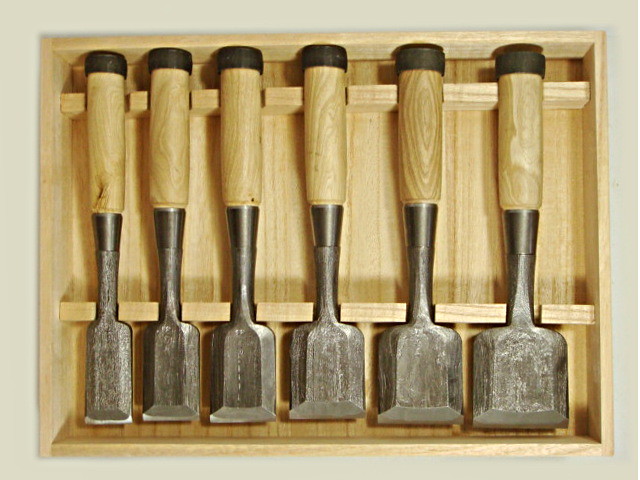The image depicts a color photograph taken from directly above an open wooden storage box made of light beige wood, showcasing its visible grain. Inside the box are six tools with wooden handles, each fitted into its built-in space within the box. The tools, presumed to be woodworking chisels of varying sizes, are arranged vertically with their metal ends pointing downward. The tools progressively increase in size from left to right, with three smaller ones on the left and three larger ones on the right. Each tool has a darker slice of wood at the tip of their handles, matching the wood of the box in color. The box itself casts a slight shadow on a beige surface below it.